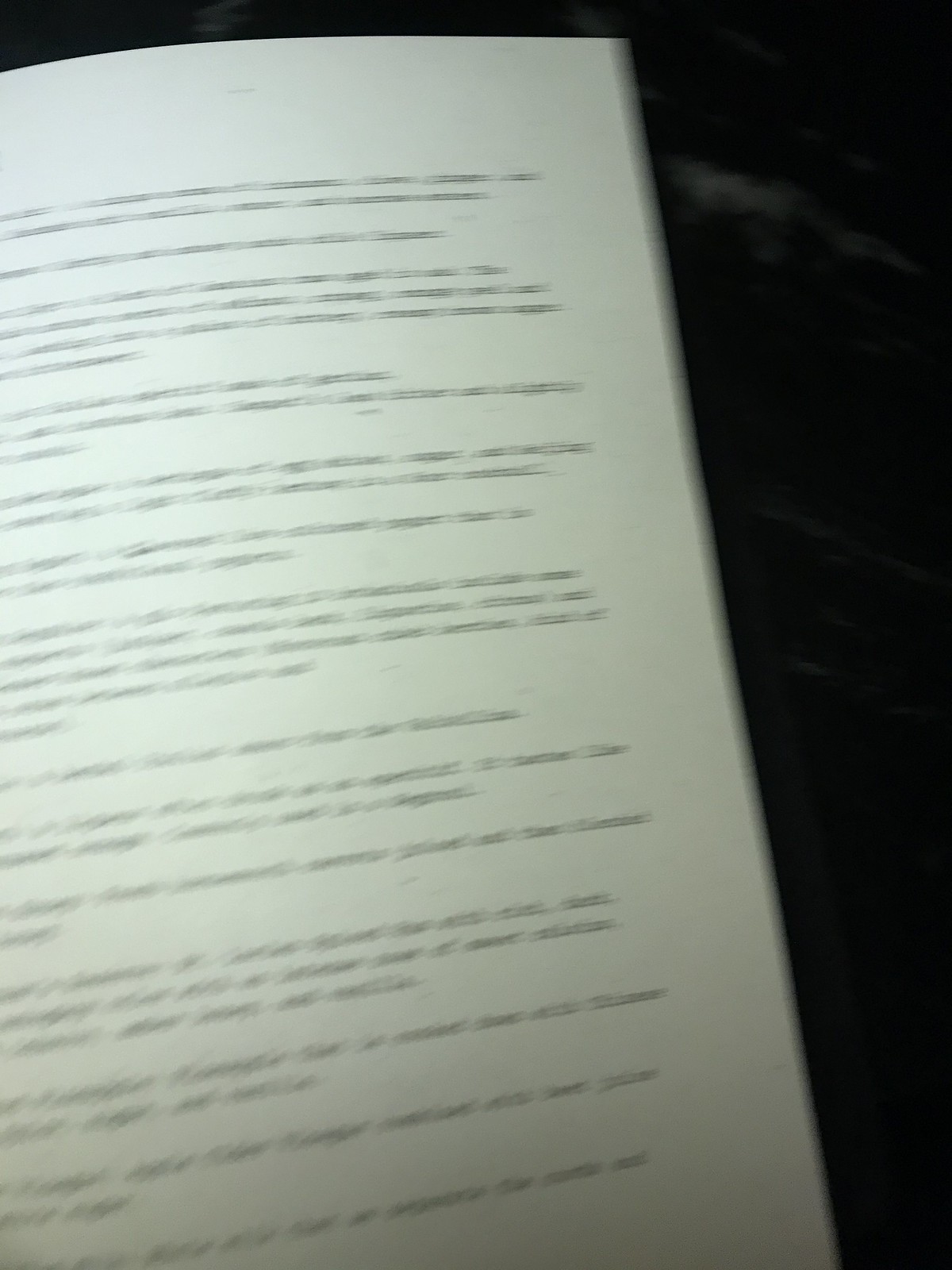This is a color photograph that is very blurry and out of focus, likely depicting a page from a book or a single printed sheet. The page takes up approximately seven-eighths of the image and is a light grayish-white. It has multiple lines of black text running from the top to the bottom, which are arranged in a pattern with varying numbers of lines interspersed with spaces. Due to the blurriness, the small black text is not readable. The top and top right of the image feature a very dark, almost black background that might be a wall or a surface, and this background has some white areas, possibly resembling a black and white marble table.